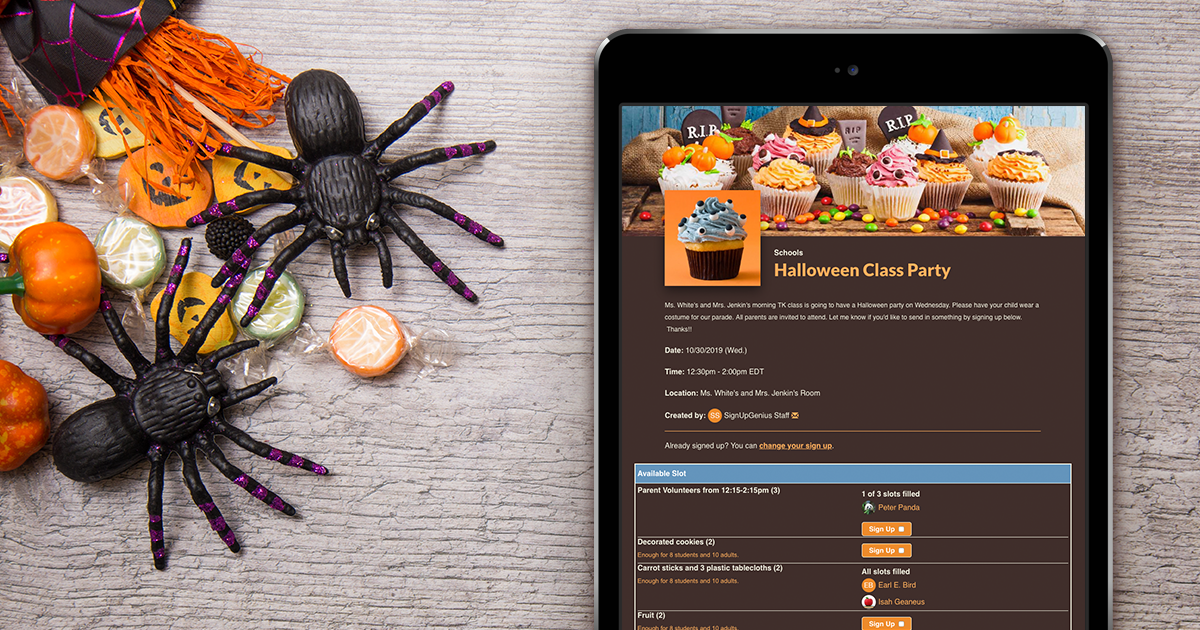A photograph captures an iPad resting on a wooden table adorned with Halloween decorations to the left. The festive arrangement includes a couple of black rubber spiders, several small pumpkins, and paper streamers, among other seasonal adornments. Scattered around are various pieces of round candy wrapped in plastic twist wrappers, adding to the Halloween spirit.

On the iPad screen, a detailed and colorful invitation to a "Halloween Class Party" is prominently displayed. The top image showcases Halloween-themed cupcakes, with one featured cupcake overlaying the profile picture area. This cupcake is striking with a blue frosting adorned with black and white dots, set in a black paper base. Below the inviting image, the text reads "Halloween Class Party" in bold letters. The area beneath this contains additional information about the party's time and location, set against a medium brown background, although the details are too small to decipher.

Scrolling down slightly, the screen reveals several segmented fields denoted as "Available Slot," suggesting a sign-up mechanism for different time slots. Each segment likely corresponds to different times or locations for the event, a feature underscored by the appearance of orange buttons designed for selecting a preferred time slot. This layout indicates the party might occur multiple times over one or several days. The entire setup on the iPad screen is clear and user-friendly, complementing the festive scene on the table.